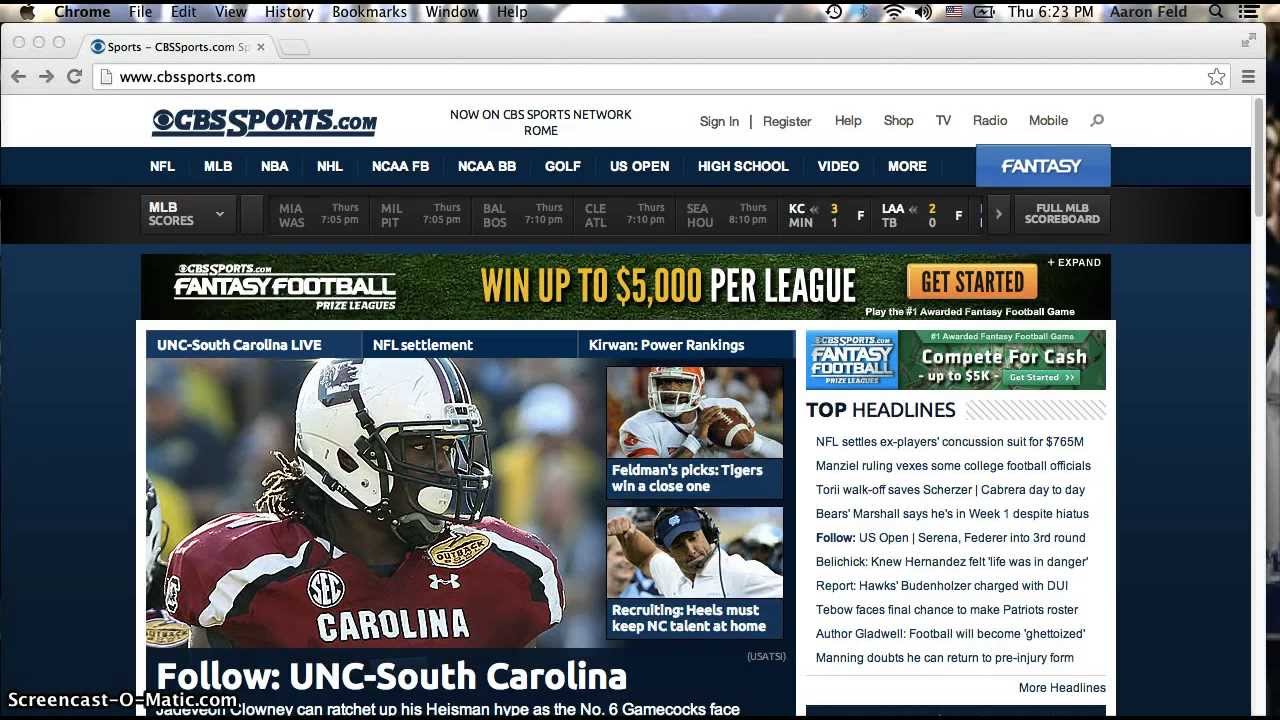Here is a cleaned-up and detailed caption based on the provided description:

---

The screenshot captures the user interface of a web browser on a macOS system, prominently displaying the menu bar and an active browser window. 

At the very top of the screen, the macOS menu bar is visible with text displayed in black. On the left, it shows the Apple icon, followed by the menu options: "Chrome," "File," "Edit," "View," "History," "Bookmarks," "Window," and "Help." To the right side of the menu bar, there are a few status indicators including an American flag icon, a Wi-Fi icon, the day and time as "THU," indicating Thursday, and the local time "6:23 PM in Ehrenfeld." Lastly, a black magnifying glass icon signifies the Spotlight search function.

Below the menu bar, a single browser tab is open and highlighted in gray. The tab displays the blue CBS logo followed by the text "sports-cbssports.com" in black. To the left of the tab, there are navigation arrows colored in gray for moving left, right, and refreshing the page. The URL bar shows "www.cbssports.com" in black text.

In the browser's main content area, the background turns white, with "cbssports.com" displayed prominently in blue text, alongside the current program "Now on CBS Sports Network, Rome" in black. Below this header, there are several navigation tabs in black text providing various options including "Sign In," "Register," "Help," "Shop," "TV," "Radio," and "Mobile." 

Another horizontal navigation menu is located beneath, set against a blue background. This menu features various sports categories labeled in white text: "NFL," "MLB," "NBA," "NHL," "NCAA FB," "NCAA BB," "Golf," "US Open," "High School," "Video," and "More." A special tab labeled "Fantasy" is highlighted in light blue.

Further down, the page shows the "MLB scores" section, displaying different team abbreviations and matchups including MIA, Washington, MILPIT, BAL, BOS, CAL, ATL, SEA, HU, HOU, KC, MINLA, and ATB.